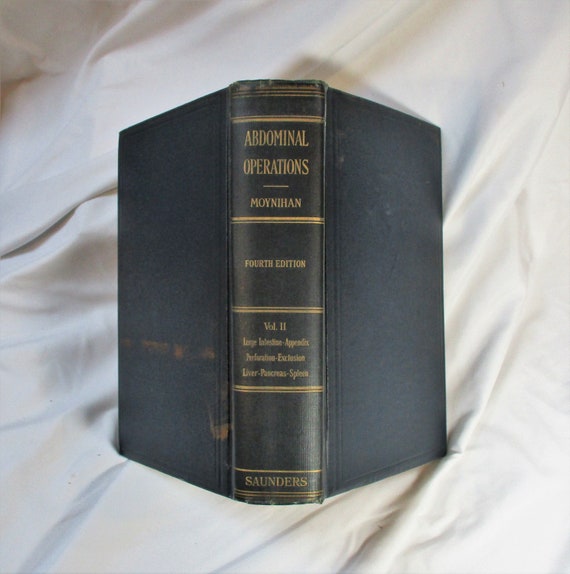The color photograph, staged and illuminated by artificial light, captures a vertically rectangular hardcover book lying open face down on a somewhat crinkled white sheet. The sheet serves as a soft and undulating background, filled with pockets of air. The book, predominantly black with no visible text on its blank front and back covers, prominently displays the intricate gold lettering and bands on its spine. At the very top, a triple gold band is followed by a double gold band. Below these bands, the spine reads "Abdominal Operations" in capital gold letters, followed by the name "Moynihan." Subsequent to another gold band, the text "Fourth Edition" appears, and beneath it, "Volume Two," along with additional smaller text that is too indistinct to decipher. Near the bottom, another gold band precedes the word "Saunders" in capital letters, concluded with an additional double gold band. This detailed text suggests that the book is likely a medical reference on surgical procedures, meant for use by doctors or surgeons.